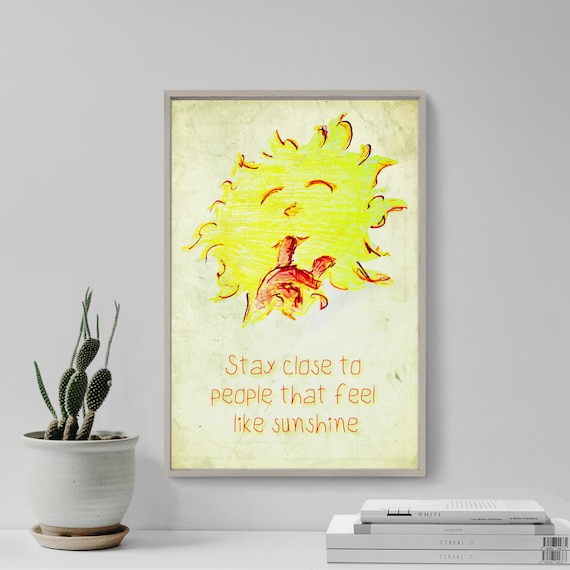In this indoor scene, a sleek gray countertop against a light gray wall serves as a minimalist stage for a thoughtfully arranged collection of items. On the left side of the countertop, a white clay pot with a tan bottom houses a vibrant cactus with four main paddle-like leaves. To the right, a neat stack of four white books—two larger ones topped by two smaller ones—lies with their spines facing outward. Mounted on the wall above the countertop is a rectangular framed picture with a thin gray border. The picture features a cheerful yellow sun with closed eyes and a raised hand, almost in a "shh" gesture, accompanied by an uplifting message: "Stay close to people that feel like sunshine," presented in an orange font. The overall scene radiates a sense of calm and positivity.